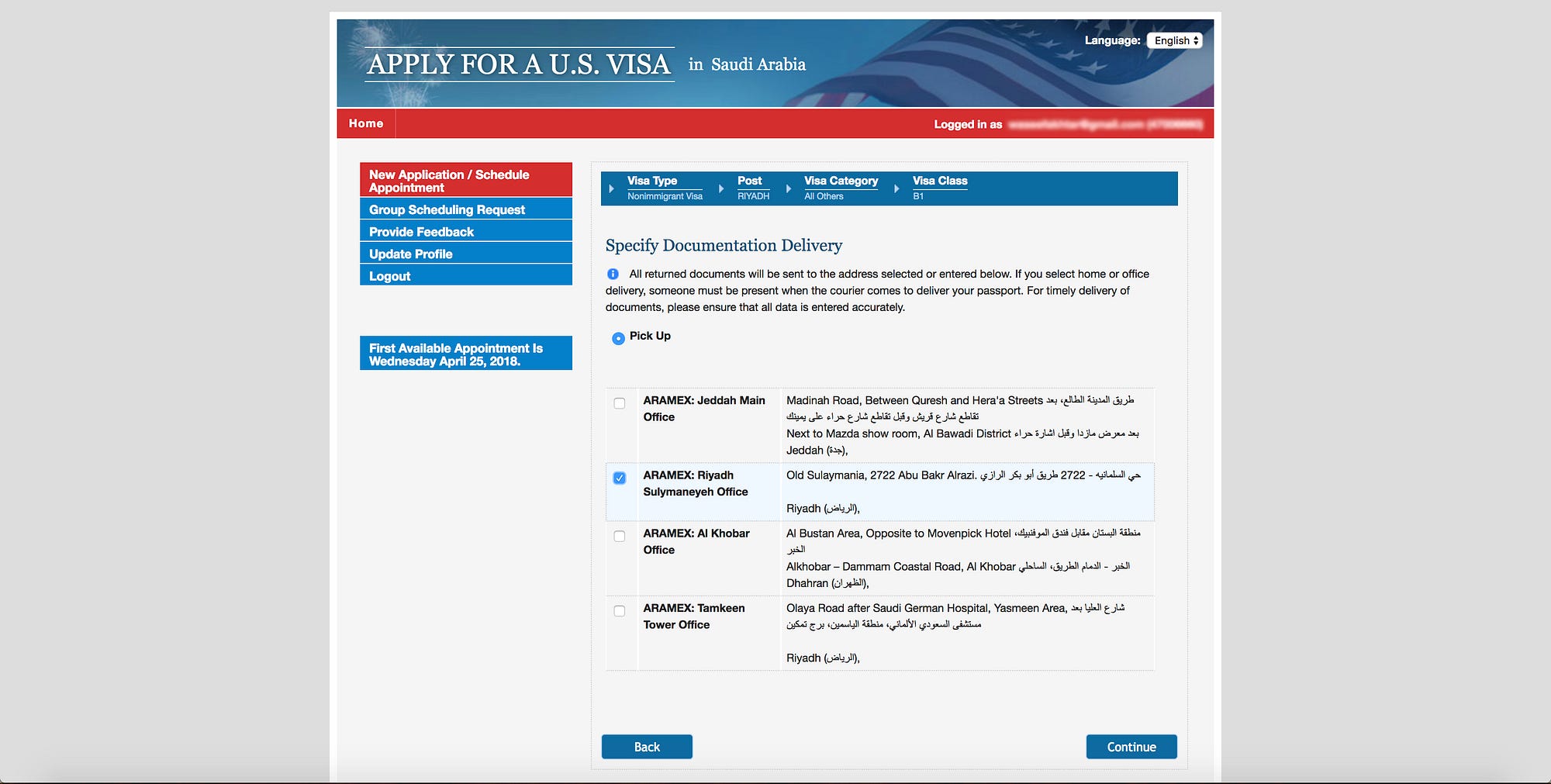This image depicts the homepage of the "Apply for a U.S. Visa" website, identifiable by its title prominently displayed on the upper bar. The upper bar features a segment of the American flag emerging from the lower right-hand corner, symbolizing the U.S. The title "Apply for a U.S. Visa" is clearly written, with "in Saudi Arabia" appearing in smaller, white font just to the right. Below the title bar, a red navigation bar spans the width of the page. On the left side of this red bar, the word "Home" is visible, while on the right side, it reads "Logged in as," followed by redacted user information.

The main content area of the website is divided into two parts. On the left side, there is a vertical menu of blue bars. The topmost bar in this menu reads "New Application / Schedule Appointment." On the right side of the main window, there is a section titled "Specified Documentation Delivery," indicating a focus on documentation procedures. The website layout suggests a structured and user-friendly approach to navigating visa application processes.